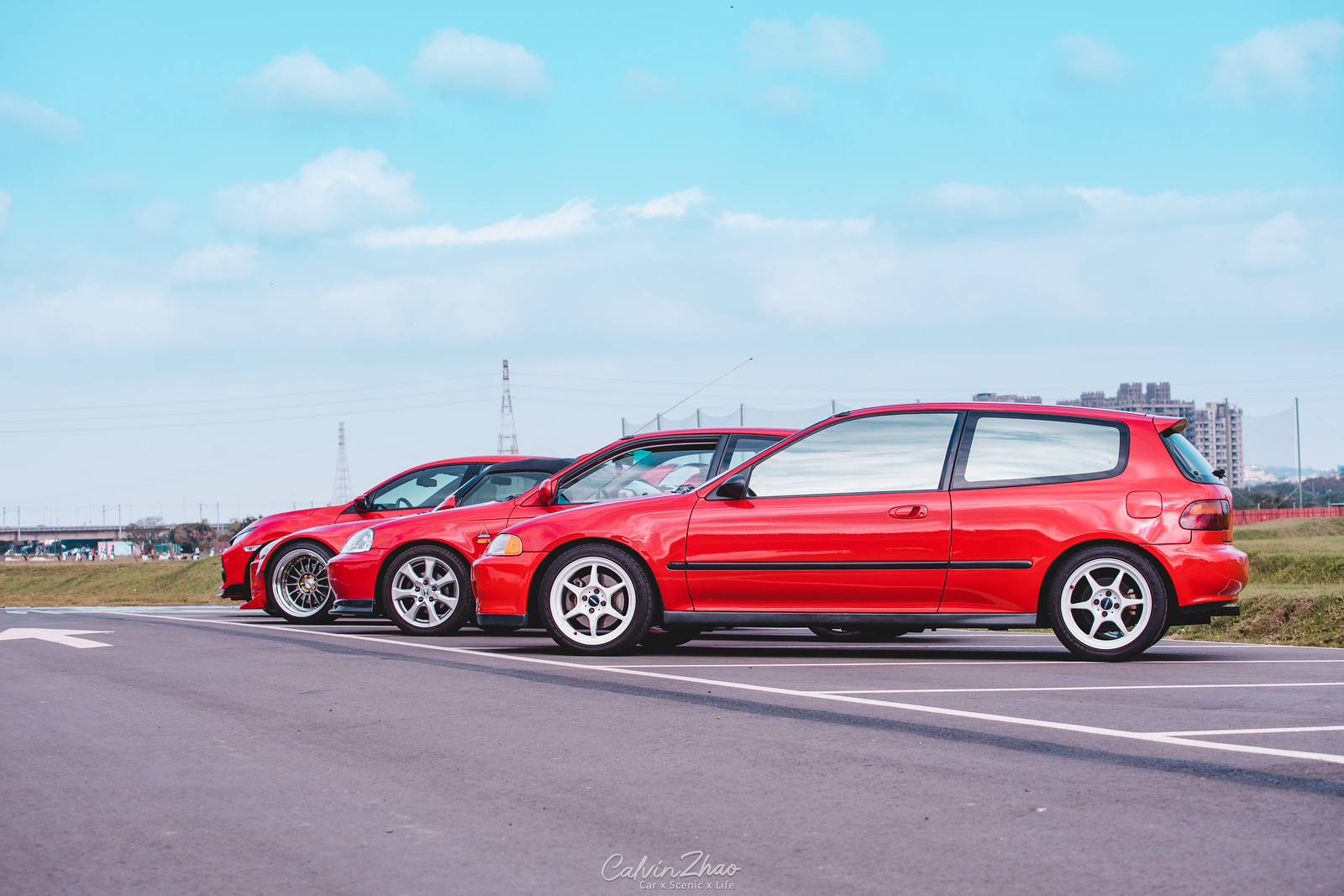In a professionally captured photograph signed by Calvin Zao (Z-H-A-O), four polished red cars are parked diagonally along a paved roadway. The vehicles, positioned in a designated parking area to the right of the pavement, all face the same direction towards the left, where a white arrow is visible on the dark pavement. Although the cars share a similar red color and aesthetic, their varying body styles and wheel structures suggest that they are not identical makes. The nearest car, a two-door with a black plastic bumper and reflective windows, stands out in the foreground, while the adjacent car features clear windows. Further back, two sportier models can be seen, each with distinctive hood lengths indicating their unique designs. The scene is set against a backdrop of tall buildings, light poles, and an overpass highway under a partly cloudy sky, evoking a sense of urban sophistication. The well-composed image, possibly resembling a car show, is further enriched by the visible watermark of the photographer, Calvin Zao, at the front.